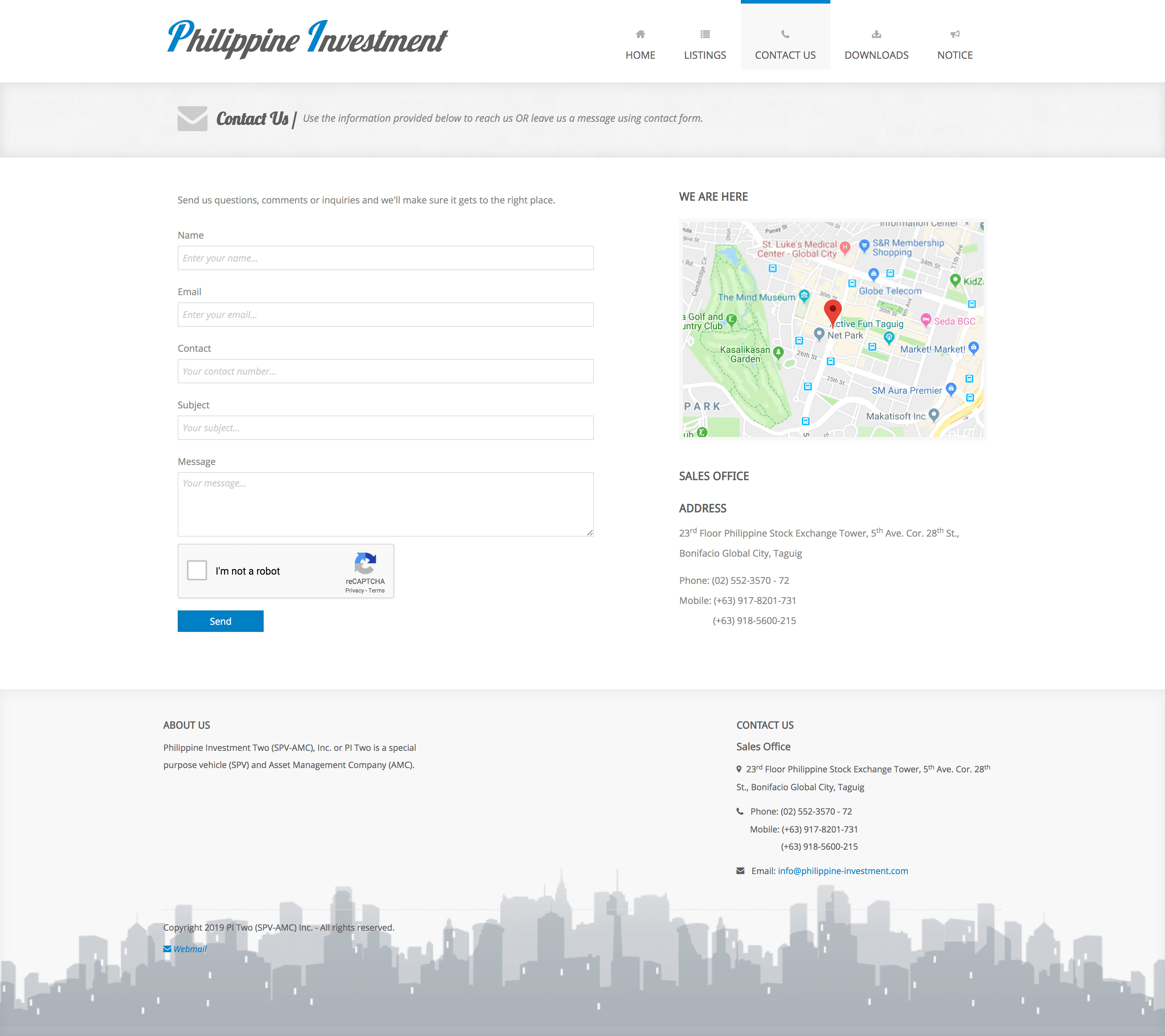The image showcases the "Philippine Investment" website against a white background. In the upper left-hand corner, the text "Philippine Investment" is displayed, with the initials 'P' and 'I' in blue, and the rest of the text in bold black font. Adjacent to this title are the navigation options: Home, Listings, Contact Us, Downloads, and Notice.

A gray-bordered section labeled "Contact Us" invites users to either reach out using the provided information or leave a message through a contact form. The white-background form includes fields for Name, Email, Contact Number, Subject, and Message, with the instructions to "Send Us Questions, Comments, or Inquiries, and we will make sure it gets to the right place." Beneath the form fields, there's a Recaptcha checkbox stating "I'm not a robot" and a blue "Send" button.

On the right-hand side of the webpage, there's a section titled "We Are Here," featuring a small map marked with a red dot to indicate the location. Below this, the Sales Office Address is detailed: 

23rd floor, Philippine Stock Exchange Tower, 5th Avenue, COR 28th Street, Bonifacio Global City, Taguig.

Contacts:
- Phone: 02-552-3570-72
- Mobile: 63917820-731

Additionally, the section reiterates the contact numbers and includes the email address Info@Philippine-Investment.com for further inquiries.